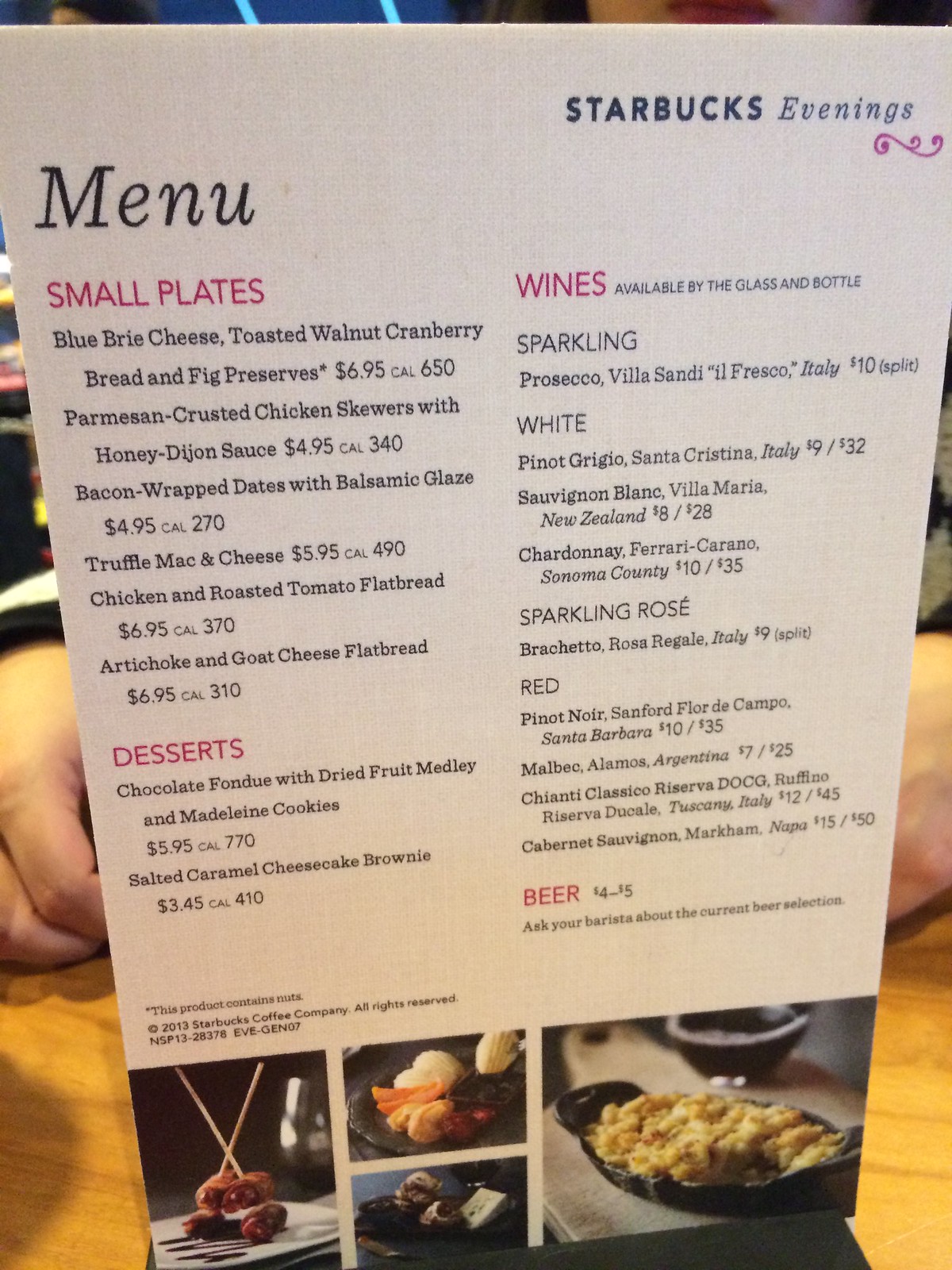This picture captures a detailed view of a Starbucks Evenings menu poised on a table. The upper right corner of the menu prominently features the "Starbucks Evenings" heading. The menu layout is divided into sections, hinting at a more varied selection than the typical Starbucks offerings.

On the left side of the menu, labeled "Menu," there is a section highlighted in red titled "Small Plates," listing several food items:
1. Blueberry cheese, toasted walnut, cranberry bread, and fig preserves - priced at $6.95.

Following the small plates, there's another section in red titled "Desserts." The highlighted dessert item is:
1. Chocolate fondue with a dried fruit medley and Medellin cookies - priced at $5.95.

The right side of the menu comprises another column starting with the title "Wines." The wine list includes categories like sparkling and white wine, sparkling rosé, and red wine. At the very bottom of the right column, the word "Beer" is written in red, with a single type of beer listed below it.

To enhance the visual appeal and help customers make informed choices, the bottom of the menu features four pictures showcasing some of the food entrées offered. These images provide a clear and appetizing preview of the dishes available, ensuring customers know exactly what to expect.